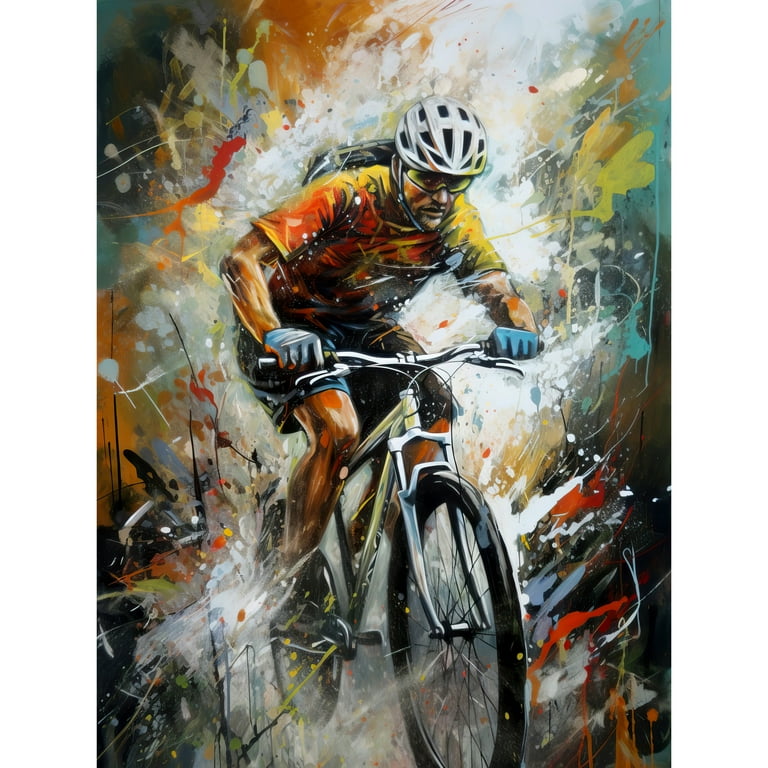This dynamic and vibrant painting portrays a bicyclist racing toward the viewer with an energetic and lively atmosphere. The cyclist, a man wearing a yellow-orange splattered t-shirt, blue pants, and black shoes, is gripping the white bike's handlebars tightly and leaning forward with intensity. He is equipped with a white protective helmet, goggles, bluish-white gloves, and a black backpack. His determined gaze is directed at the viewer, adding to the thrilling sense of motion. Surrounding him is a multicolored explosion of paint splotches—prominently featuring white, red, yellow, orange, and blue—which creates an impression of movement and excitement, almost as if he is bursting through the canvas. The faint orange and black undertones in the background add depth to this action-packed scene, suggesting either a manually painted masterpiece or a sophisticated computer-generated image that captures the essence of speed and color.